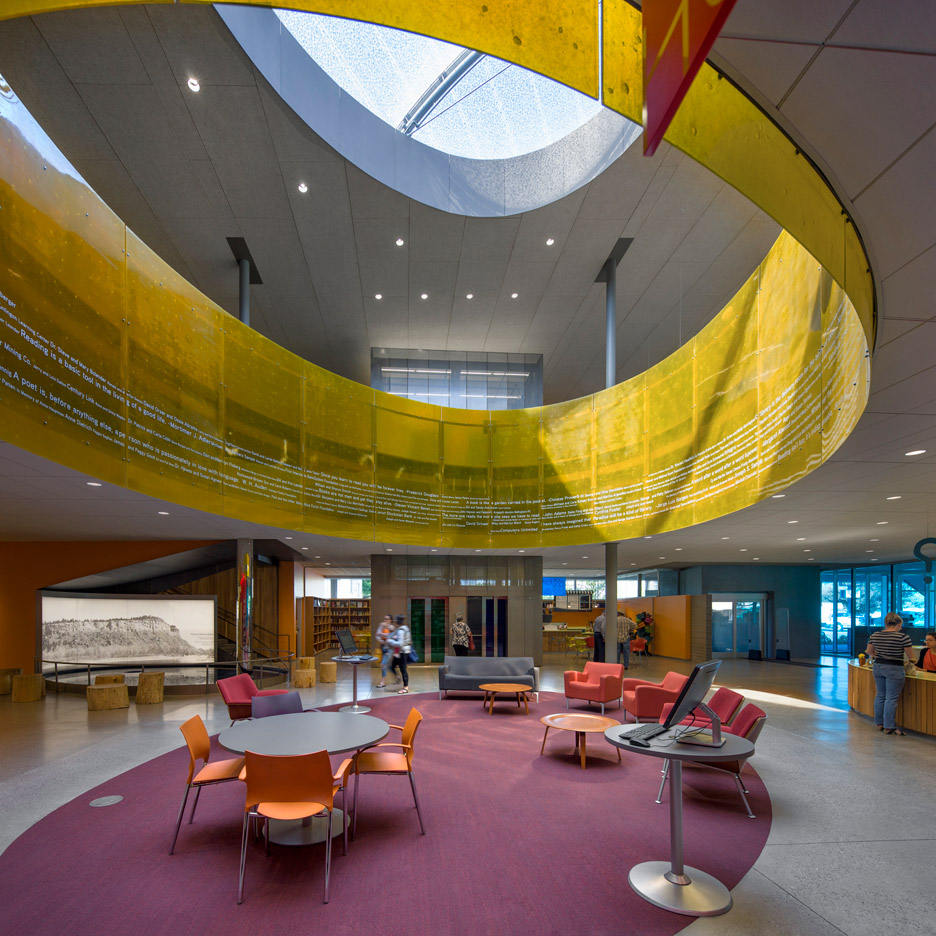The image captures the interior of a large, well-lit public building, likely a college library or student center. Dominating the space is a prominent skylight, which allows natural sunlight to flood in, casting a warm glow on the scene. Directly beneath the skylight, a striking yellow circular structure with a railing encloses an upper-level walkway where five or six people are casually strolling.

The central area is furnished with a mix of colorful seating arrangements: gray couches, pinkish armchairs, and orange and red chairs, all situated around various circular tables. A noticeable purple oval rug anchors the space, adding a splash of color. In the foreground, there's a tall stand equipped with a computer and keyboard, likely for student use. 

Further back, one can see a desk to the right where a woman is conversing with a receptionist or librarian. This area seems to function as an information or checkout desk. To the far right, there is a hint of brown library shelves, solidifying the setting as a library. The background shows more people in motion, including one student in a striped shirt and jeans, adding a touch of dynamism to the serene setting. Additionally, there are indications of elevators or doors and possibly a large screen displaying information.